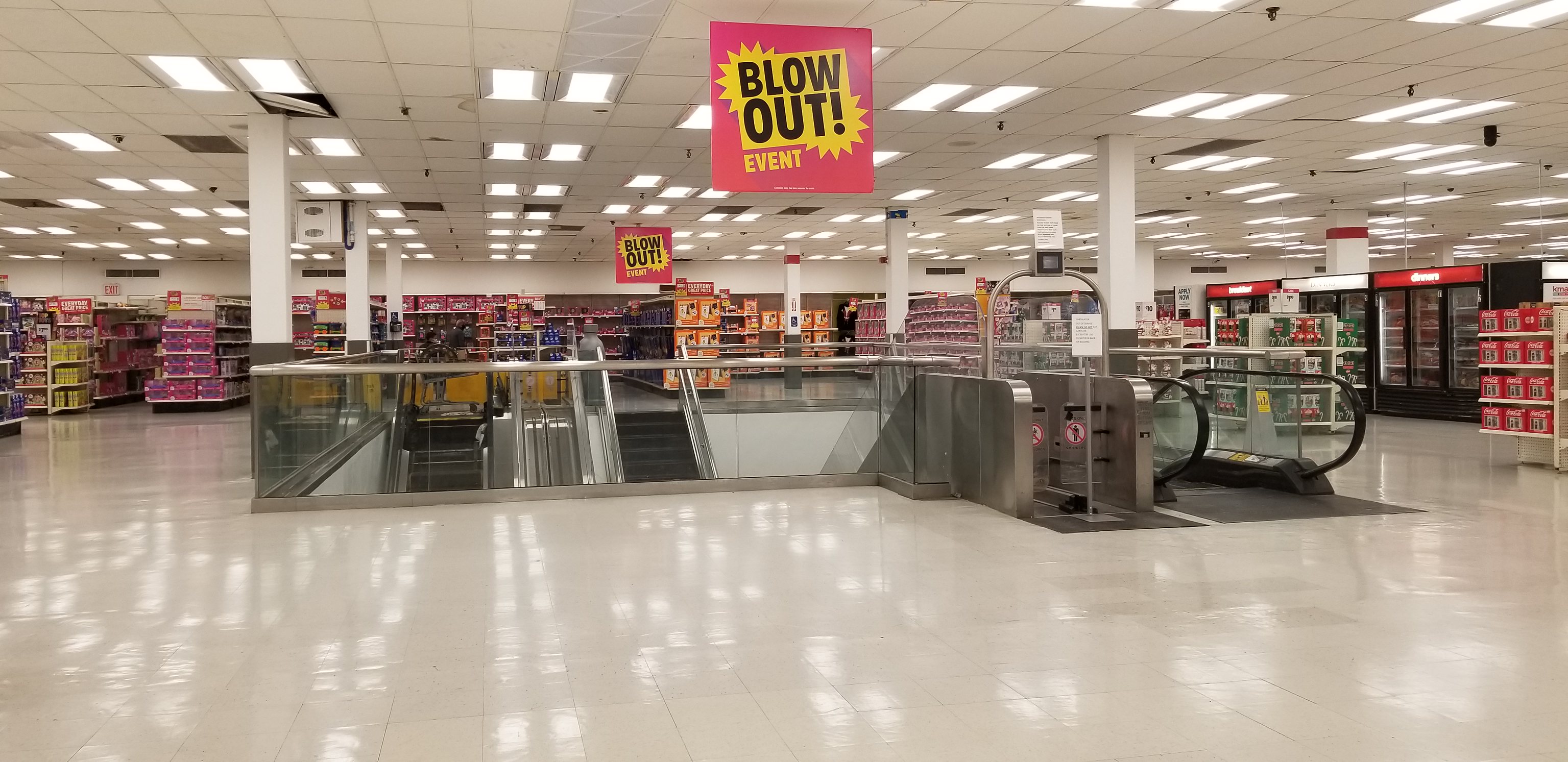The image depicts the interior of a bustling retail area where a large sale event is taking place. Dominating the scene is a prominent square sign suspended from the gray-tiled ceiling, featuring the words "Blowout Event" in bold black text against a vivid red and yellow background. The gleaming white tiled floor reflects the rows of square lights above, adding to the store's bright ambiance. In the foreground, two black-stepped escalators, trimmed with transparent glass and chrome barriers for safety, provide access to different store levels. To the left of the escalators, stacks of what appear to be toys are visible, hinting at a toy department. Meanwhile, red signs on the right proclaim "Everyday Great Price." Several rows of stocked shelves stretch into the background, their contents indistinct but hinting at a variety of merchandise. White columns punctuate the store's layout, adding structural elegance to the extensive retail space.